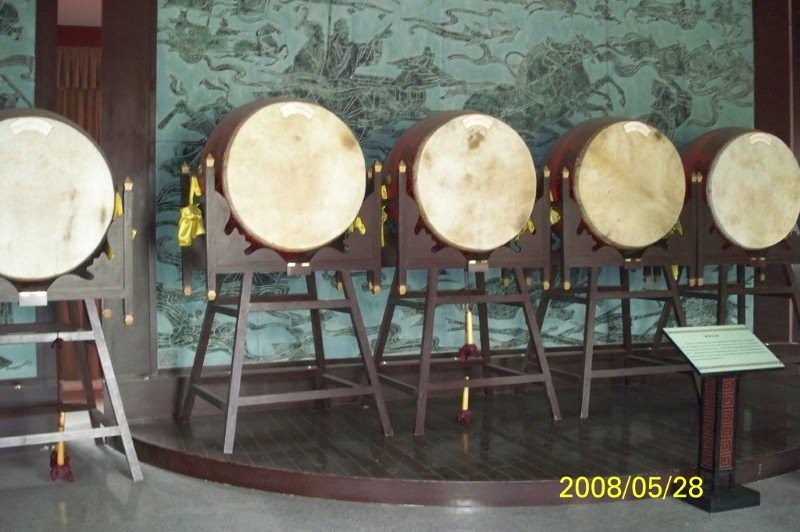The photograph captures a display of several drum-like objects with a bear-like appearance, showcased as part of an art exhibition or museum display. Each drum features a mottled white and tan membrane stretched over its surface, facing the camera. They are securely positioned inside elaborately carved wooden cradles, which possess gold decorative tips on their corner posts. These stands rest on a short, raised stage made of dark, shiny wood planks. The backdrop consists of a light green wallpaper or mural, adorned with dark green figures depicting people and horses, suggesting an Asian influence. A small sign with illegible writing is visible in the lower right-hand corner, along with a date stamp reading "2008-05-28." This setting suggests a meticulous presentation, possibly narrating the historical or cultural significance of the instruments.